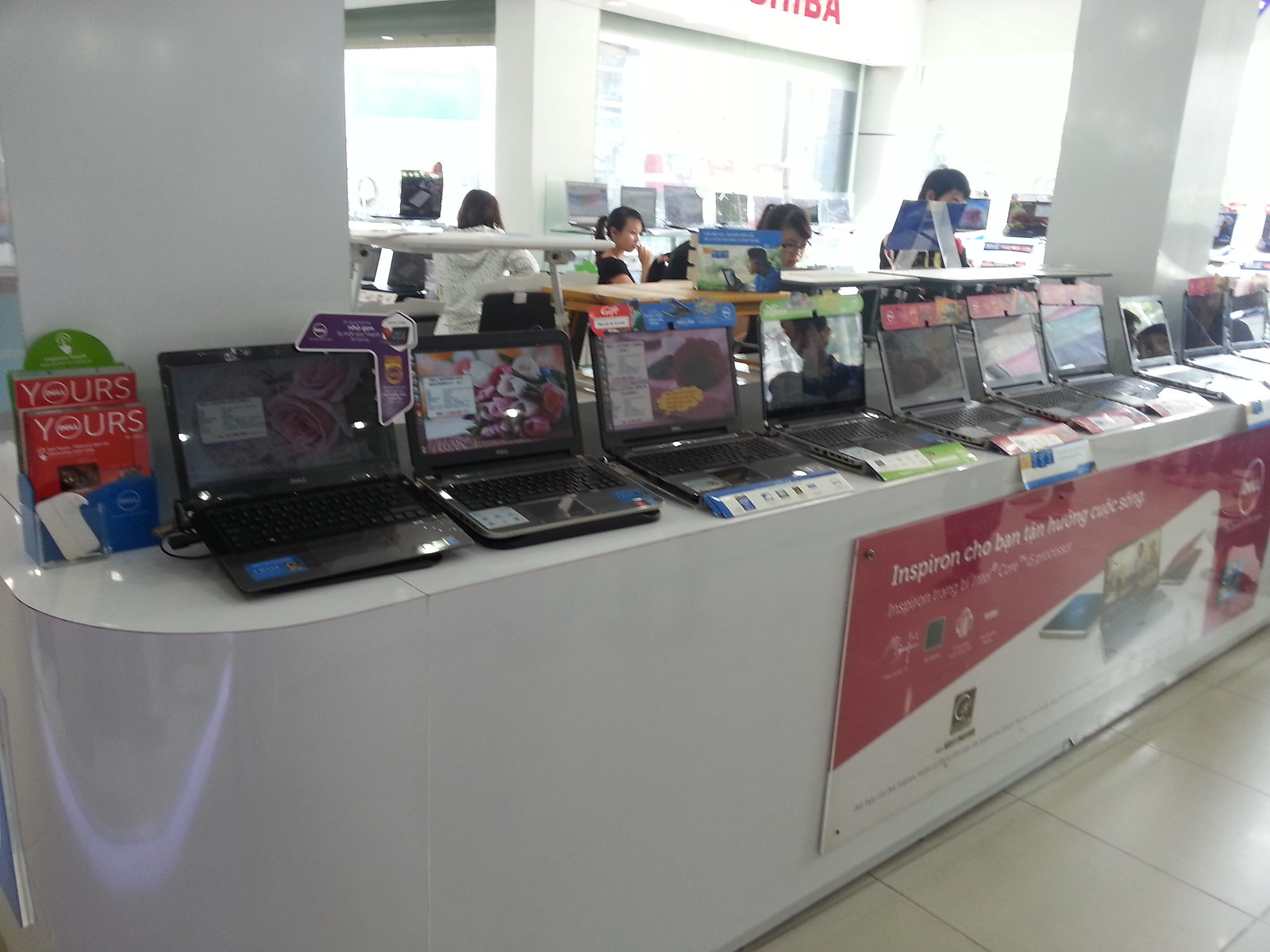The photograph, taken indoors, showcases an electronic store specializing in laptops. At the forefront, there's a solid white display table draped in white cloth, likely plastic, featuring ten open laptops facing the camera. The screens display various content, though it's not clearly discernible. Scattered across the table are brochures and a distinctive red and white magazine titled "Yours" with laptop images on its cover. Above, a red Toshiba logo adorns the wall. The store's interior is predominantly white with off-white tile flooring. Three thick, square white columns are visible, with one prominently positioned in the upper right and another on the left. People are seen browsing and examining the laptops and other products. Some laptops have colorful cardboard tags indicating different features, and banners with the word "Inspiron" drape the sides of the table. The overall ambiance is bright, spacious, and neatly organized, focusing on the display and sale of laptop computers.